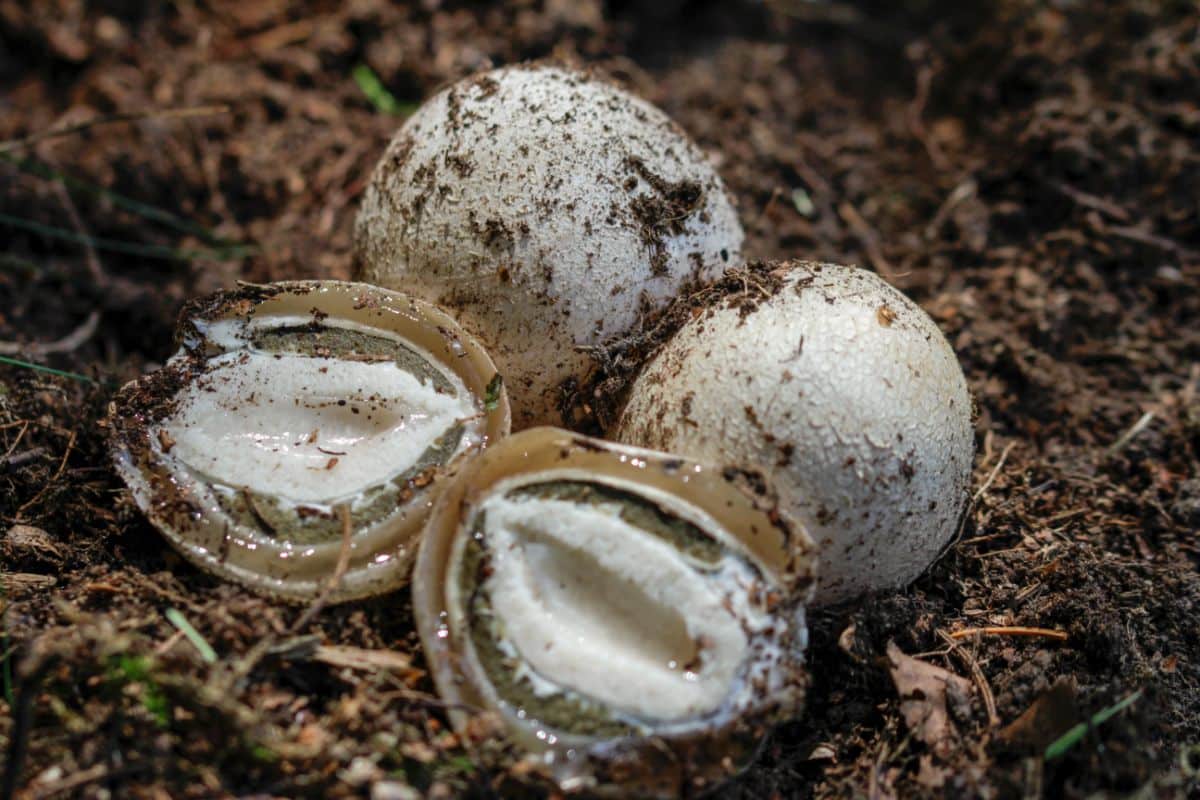The image captures a close-up of four round, white objects nestled together on a dirt ground, likely in a forest setting. The foreground shows a mix of soils, plant debris, and small pieces of wood. These objects resemble eggs or fruit but might also be white mushrooms. Two whole pieces are intact, while two are cracked open, revealing their interiors. The opened objects display a firm, white inside without any yolk, surrounded by a dark brown perimeter. The surface of these objects is slightly dirty due to their contact with the earthy surroundings. The scene is detailed and gives a sense of an undisturbed natural habitat.